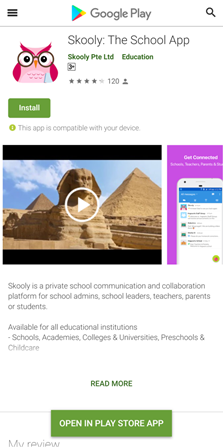This is a detailed and descriptive caption for the image:

---

This is a screenshot taken from the Google Play Store on a mobile device, evident from its rectangular shape. The background is white, giving it a clean and minimalist appearance. 

At the top left corner, there are three horizontal black lines, stacked one above the other, serving as the menu icon. On the top right corner, there is a black search icon, typical of the Google interface. Centrally positioned, the iconic sideways triangle emblem of Google Play is displayed, colored in blue with a touch of yellow at the tip, and red at the base, followed by the "Google Play" text in black font. Beneath this central header, a thin gray line delineates the start of the app listing section.

On the left side of the app section, there's an image of a pink owl with black glasses, staring directly at the viewer with a slight scowl. Adjacent to this owl, towards the right, the app name "Schooly" (spelled S-K-O-O-L-Y) is prominently displayed in bold black text, followed by the phrase "The School App" in standard black font. Below this, "Schooly P-T-E L-T-D" is listed in green text, with "Education" following after a small space, also in green. A small white square with a black border housing the age rating "3+" is noticeable beside this information.

Below the app details, the app's rating is depicted with four dark gray filled stars and one light gray star indicating a partial rating, joined by the number "120" and a small profile icon symbolizing user interactions. Directly beneath the pink owl, there is a distinct green button labeled "Install" in white text. Just below this, there is a green circled lowercase 'i' icon, next to which it states in gray font, "This app is compatible with your device."

Further down, occupying about two-thirds of the horizontal space, there is a video featuring a pyramid in Egypt, with a white play button situated at its center. The video is framed by thin black borders both at the top and bottom. On the right side of the video, a small popup purple tab appears, bearing an unclear, blurred foam design.

Below the video, there are several lines of text, with three lines followed by a space, another set of three lines followed by another space. Centrally positioned amidst the text is a green, all-capitalized button that reads "READ MORE." Approximately an inch below this button is a green tab, boldly capitalized in white text, stating "OPEN IN PLAY STORE APP."

---

This caption offers a comprehensive and organized description of the screenshot, capturing all critical visual elements and providing clear context for each component.